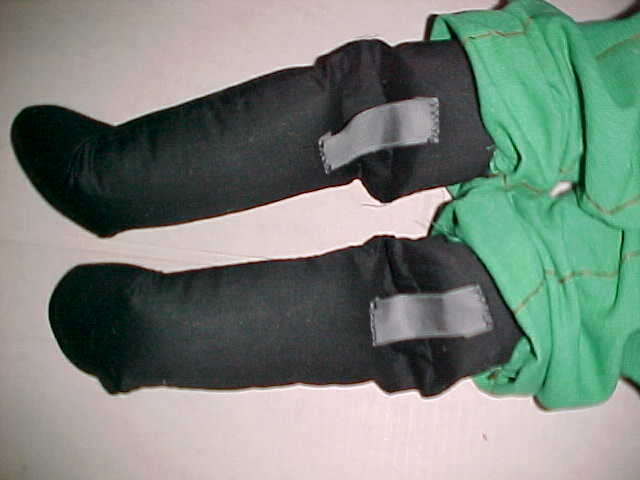The image depicts the legs of a fabric doll lying on a plain white surface, likely taken indoors. The doll's lower limbs are adorned with long, black boots that extend up to the knees. Each boot features a gray patch stitched on, with one patch located near the inner knee of the right leg and another on the front of the left leg. Above the boots, the doll is wearing green pants that appear to be crumpled or rolled up around the knees, with gold or brown lines extending vertically from bottom to top. The image itself is grainy and somewhat out of focus, adding an element of ambiguity to the details.